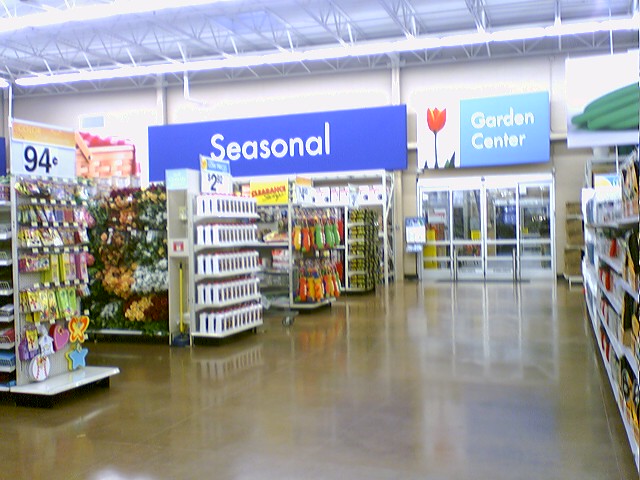This image captures the interior of a large store, resembling a Walmart, characterized by spacious, warehouse-like high ceilings and a shiny brown tile floor. Dominating the back of the image are two prominent blue signs: one reading "Seasonal" in sans serif white letters and another indicating the "Garden Center" with a red rose icon next to it. Below the garden center sign are four glass doors leading to an additional section of the store. The photo, although low quality, shows four aisles to the left, identified as part of the seasonal decor section. The nearest aisle on the left side showcases items priced at 94 cents, hanging products shaped like stars, baseballs, and hearts. Adjacent to this is another aisle featuring faux plants in greens, whites, and yellows, with a sign above pricing items at $2.62. Additionally, there's a yellow clearance sign prominently marked in red. On the right side of the image is a slightly angled aisle with a blurry depiction of what looks like part of a garden hose. The aisles display a mixture of colorful items, hinting at a summer-themed seasonal section, yet the store appears devoid of shoppers, focusing solely on the arranged merchandise.